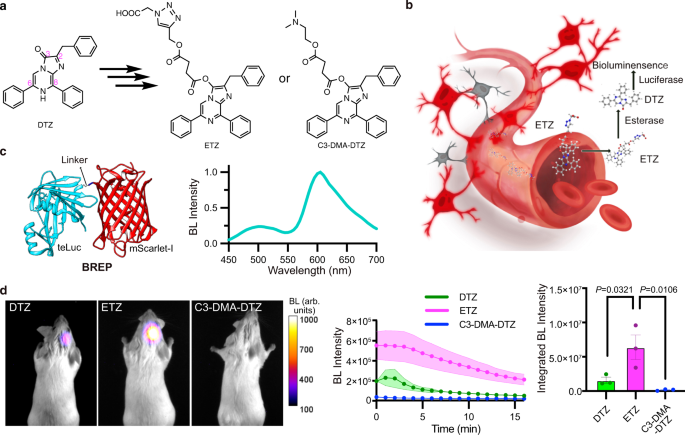The image is a detailed scientific diagram, organized in a landscape layout and divided into sections labeled A, B, C, and D. The top row features A and B, with A presenting a flowchart of molecular structures connected by arrows and annotated with letters and descriptive text. Section B details a vein-like illustration accompanied by arrows and descriptive labels, highlighting various nerve components such as bioluminescence and esterase. The middle row, labeled C, includes two illustrations resembling blue and red ribbon-like DNA strands, flanked by text, as well as a black graph labeled "BL intensity" with numerical values along the axes. The bottom row, labeled D, displays three x-ray images of a rat, prominently focusing on the brain area, followed by two colorful charts in pink, green, blue, and black hues with detailed labels. This comprehensive medical diagram encompasses various compounds, nerve structures, DNA sequences, and graphical data, meticulously arranged to convey complex scientific information without any human presence.